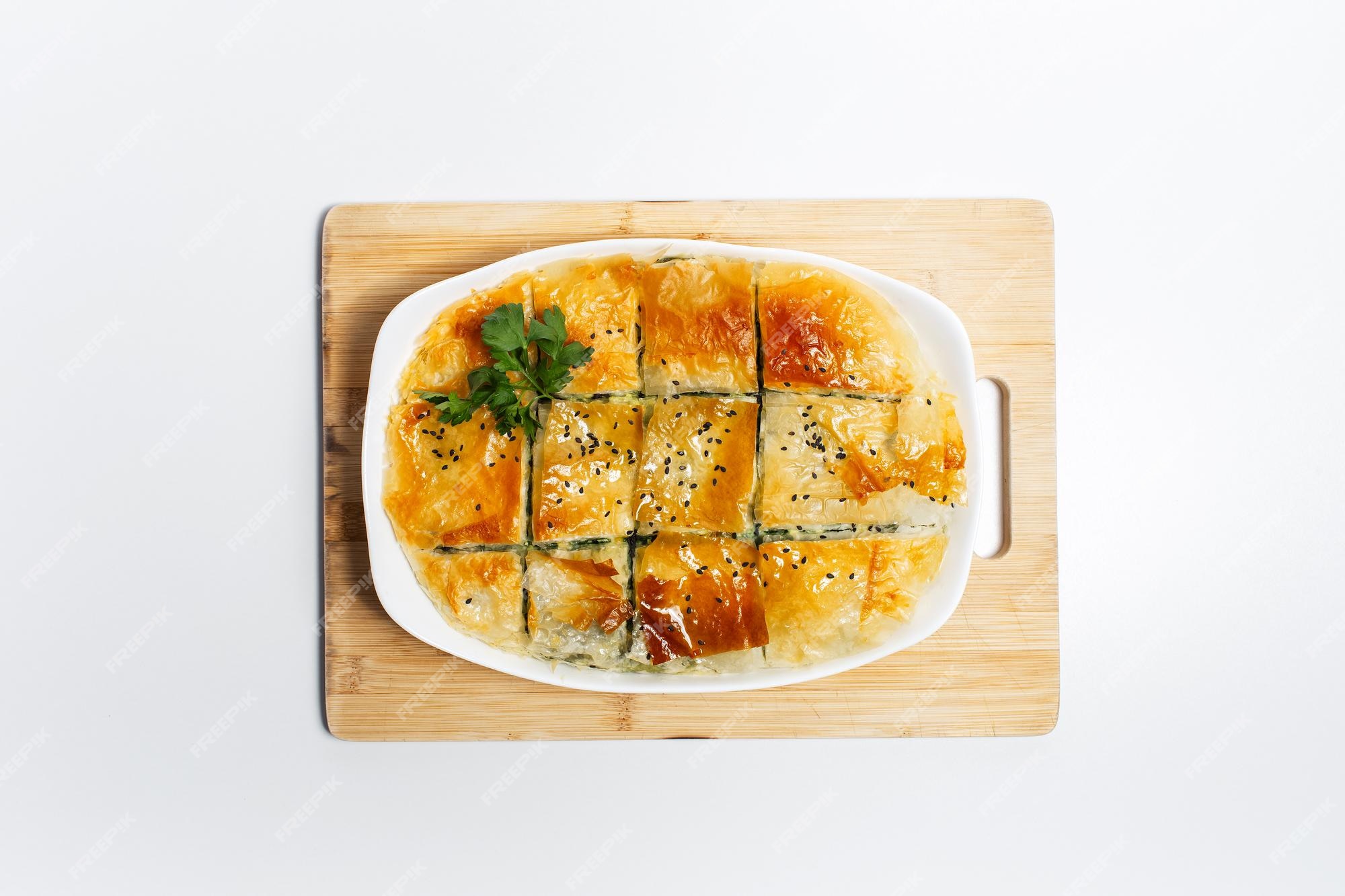The image features a delectable food dish set against a pristine white background, likely suitable for social media platforms such as Instagram or Pinterest. The central focus is a wooden cutting board, atop which rests a white serving platter containing a visually appealing dish. The dish appears to be a type of flaky breakfast pastry or Asian-inspired dish with a perfectly golden-brown phyllo or pie-like crust. The top is adorned with a scattering of sesame or black seeds, adding a delicate crunch.

The dish is cut into square or rectangular slices, revealing tantalizing hints of the filling within, which could include cheese and possibly spinach. A few green leaves, possibly parsley, add a touch of garnish in the top left-hand corner, enhancing the dish's visual appeal. The bird's-eye view of the photo captures the dish in all its crisp, clean, and inviting glory, making it look incredibly delicious and ready to enjoy.